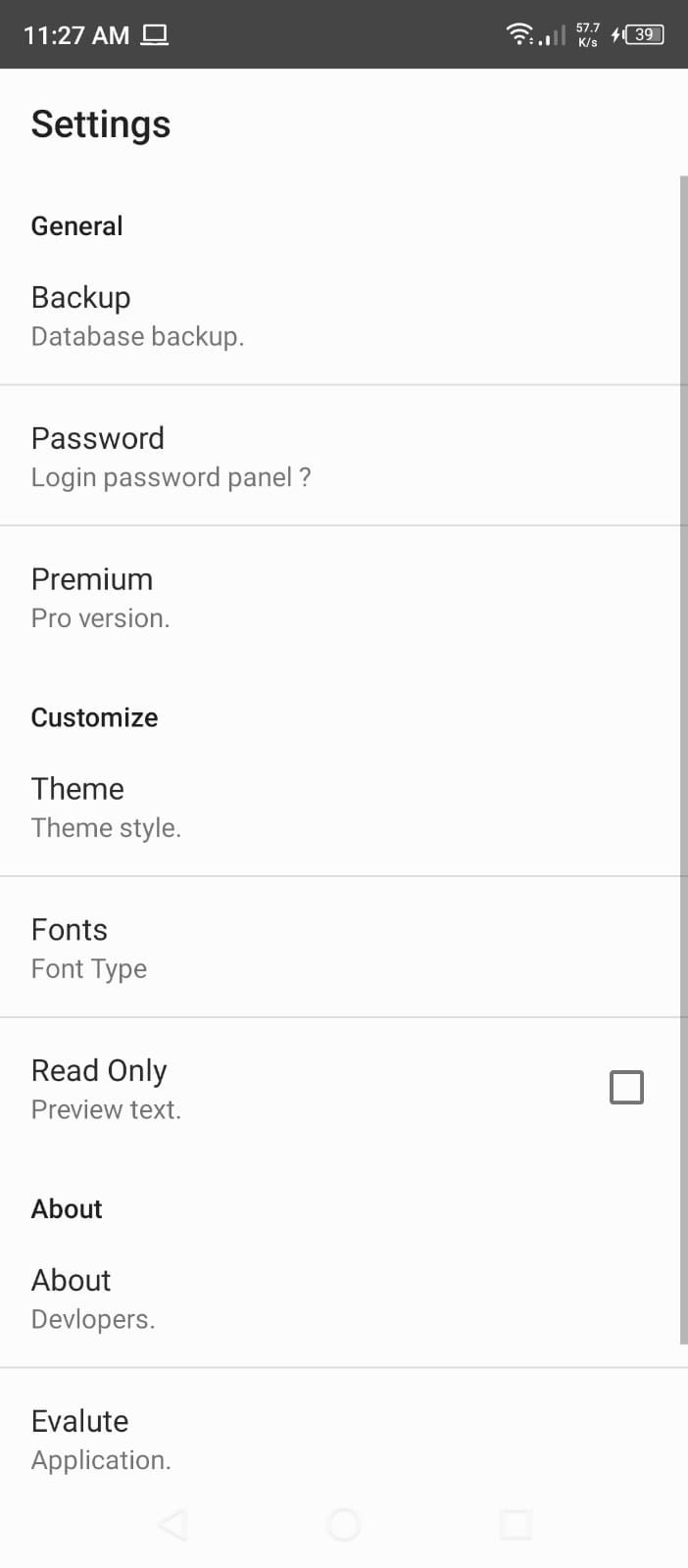The image is divided into two sections. The top portion features a black background with "11:27 AM" displayed in white text on the left side. Directly beneath is a small white rectangle, adjacent to a Wi-Fi symbol with two out of four bars filled, indicating moderate signal strength. Below this, there is white text reading "57.7 KS/S" followed by a lightning bolt icon, signifying that the device is charging, with the battery level at 39%.

The lower portion of the image transitions to a white background, beginning with the heading "Settings" in black text, followed by a list of options: "General," "Backup," and "Database Backup." A thin gray line separates each item.

The next section labeled "Password" includes the phrase "Login Password Panel?" followed by another thin gray line. Below this are options labeled "Premium" and "Pro version," followed by "Space" and "Customize." Further down, the text reads "Theme," "Theme Style," and another thin gray line.

Next is the "Fonts" section, asking, "Is this font type?" This is followed by a gray line. The subsequent entries are "Read Only," "Preview Text," "About," and "About Developers." Another thin gray line separates "About Developers," which is punctuated with a period. 

The final part of the image includes "Evaluate" followed by "Application," with each word clearly spelled out (A-P-P-L-I-C-A-T-I-O-N) and ending with a period.